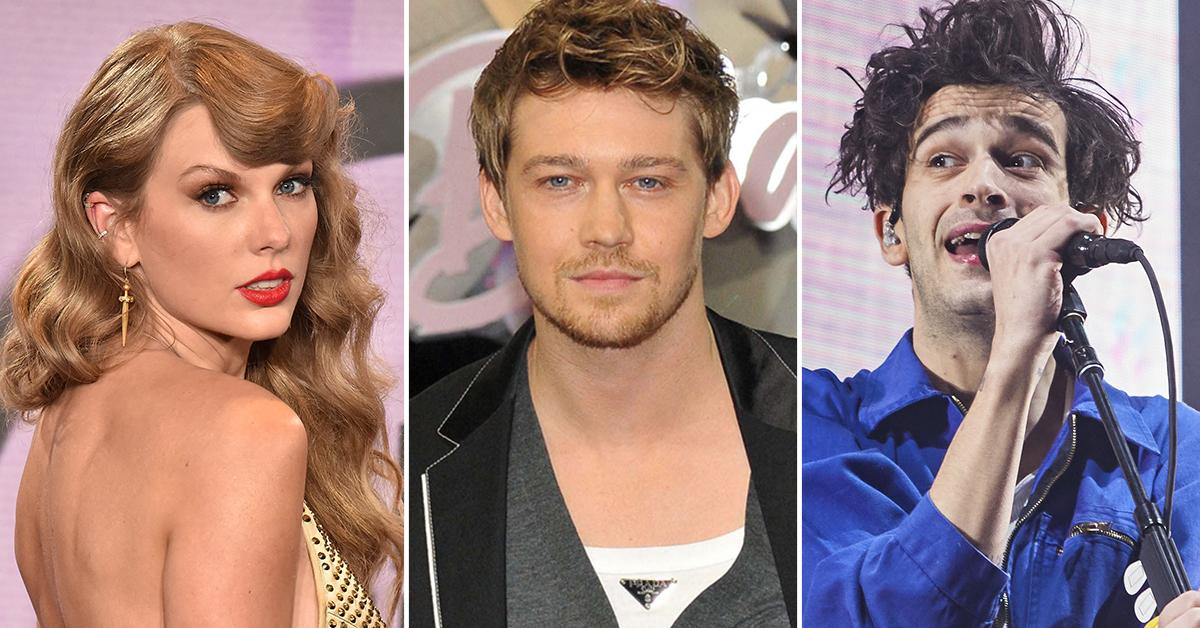The image consists of three evenly sized and spaced photographs arranged side by side. Each photograph is separated by a thin vertical line. The left photograph features Taylor Swift against a purple or pink background. She is dressed in a backless, yellow halter top with gold studs, wearing gold pointy earrings, and sporting reddish blonde hair. Taylor's right shoulder is bare as she turns to look over it towards the camera, showcasing her blue eyes and signature red lipstick. 

The center photograph shows a male celebrity who is believed to be one of Taylor Swift's former boyfriends, though his name is not specified. He stands in front of a marquee that reads "Barbie," and has short, tousled, dirty blonde hair with light highlights. He has blue eyes, a faint goatee, consisting of a light mustache and chin whiskers, and is dressed in a black jacket over a gray V-neck shirt.

The photograph on the right depicts another male celebrity with wild, messy dark brown hair that sticks up and out to the sides. He is wearing a blue long-sleeved collared shirt that zips up the front. This individual is holding a microphone and singing, with his gaze directed towards the left, set against a purple and white striped background.